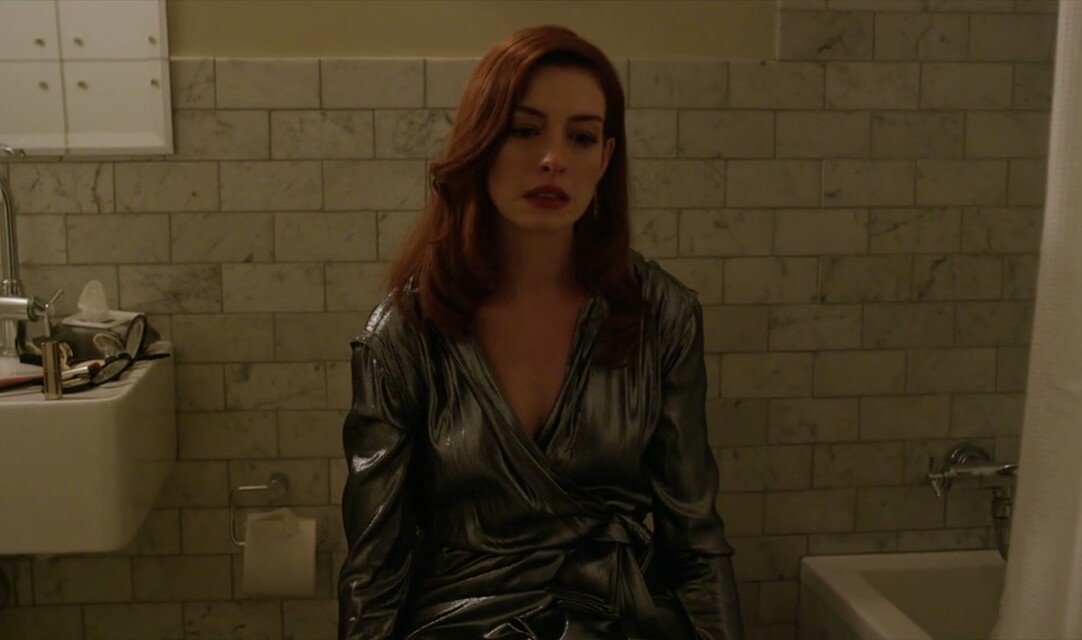In this poignant scene from a film, A-list actress Anne Hathaway is featured in a dimly lit bathroom, conveying a deep sense of despair and vulnerability. She sits on the toilet, her body nearly limp and on the verge of collapse, clutching to maintain her composure. The backdrop includes a range of bathroom elements: white tiles, a bathtub, a toilet paper roll on the wall behind her, and a sink strewn with her personal belongings. Anne is dressed for a festive occasion, wearing a glistening dress that suggests she has come from a party or special event. Her hair is distinctly red, adding to the dramatic effect of the scene. The cinematography captures the mood with a darker ambiance, enhancing the emotional weight of the moment. Despite the evident turmoil, she hasn't succumbed to tears just yet, making this a deeply moving and evocative portrayal.